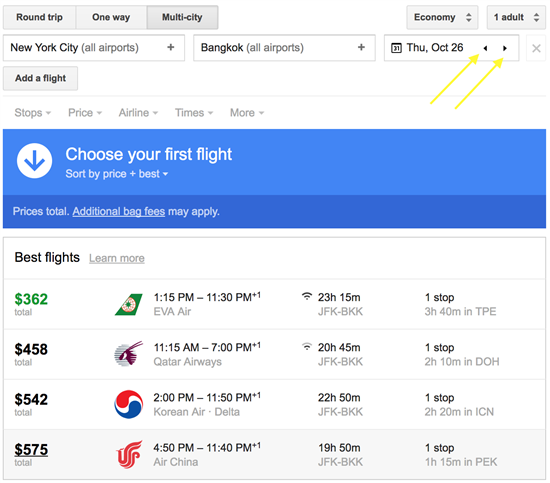The webpage displays a user-friendly interface for finding flights, starting at the top with tabs for selecting the type of trip: Round-Trip, One-Way, or Multi-City. Below the tabs, there are options to choose the travel class (Economy) and the number of passengers (one adult). The flight search details show a departure from "New York City - All Airports" and an arrival at "Bangkok - All Airports," with the travel date set for Thursday, October 26.

The interface features an option to add additional flights and provides various filters such as Stops, Price, Airline, Times, and More. A prominent horizontal blue rectangle with white text contains a drop-down arrow and the "Choose Your Flight" button, alongside sorting options like "Sort by Price + Best." Below, a darker rectangle notes that the prices listed are total costs but may include additional bag fees.

Further down, a detailed list of available flights is displayed, with prices ranging from $362 to $575, allowing users to easily compare and choose the best flight options.